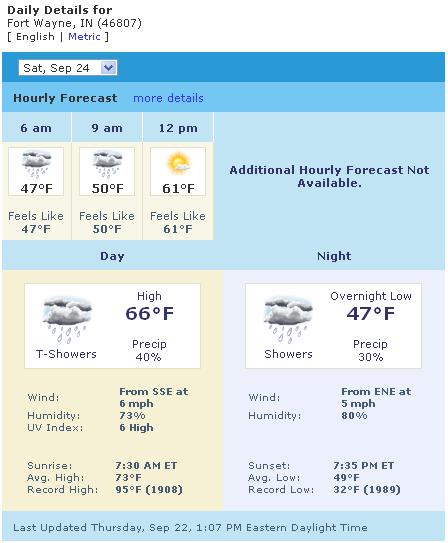This image depicts a weather website focused on providing detailed weather updates for Fort Wayne, Indiana, with the zip code 46807. At the top of the website, prominently displayed in bold black letters, is the heading "Daily Details For." The background of the website features a blue color scheme, interspersed with light gray and yellow tiles in certain areas. 

The date indicated on the website is Saturday, September 24th. A drop-down box is available for selecting different dates, and the site offers an hourly forecast feature with a "More Details" button to the right. Specific timestamps—6 a.m., 9 a.m., and 12 p.m.—are shown alongside corresponding weather icons.

An additional note mentions that if the hourly forecast is not available, other information will be provided. The forecast for the day predicts a high of 66°F with thundershowers, while the overnight low is expected to be 47°F. The weather information was last updated on Thursday, September 22nd, at 1:07 p.m. Eastern Daylight Time.